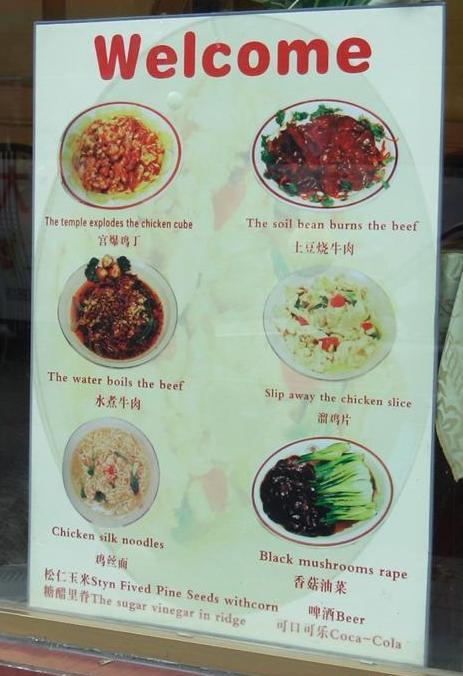Welcome Menu: 

The menu prominently features a welcoming header in bold red text. Below the header, six dishes are displayed with corresponding images, each one uniform in size and arranged in two columns.

**Top Left: "Temple Exploded Chicken Cube"** 
A tantalizing dish of well-seasoned chicken cubes, creatively named to pique interest.

**Middle Left: "Water Boils Beef"** 
This dish includes tender beef slices cooked in a savory broth.

**Bottom Left: "Chicken Silk Noodles"** 
A delicate noodle dish interwoven with thin strips of chicken, offering a harmonious and light texture.

**Top Right: "Soil Bean Burns the Beef"** 
A hearty combination of beef and beans, providing a rustic and robust flavor palette.

**Middle Right: "Slip Away Chicken Slice"** 
Thinly sliced chicken, likely prepared with a technique to keep the meat tender and juicy.

**Bottom Right: "Black Mushroom and Rape"** 
A vegetable-forward dish featuring black mushrooms and leafy greens, emphasizing earthy flavors.

Each dish name is accompanied by a corresponding image, and both English and Mandarin/Cantonese translations are provided beneath each description.

**Drink Options:**

Below the featured dishes, the menu lists drink options:

- Stein (presumably a type of beer)
- Fine Pine Seeds with Corn
- Sugar Vinegar Ridge
- Beer
- Coca-Cola

Each drink is also translated into Mandarin/Cantonese, ensuring clarity for a diverse audience.

The arrangement is neat and visually appealing, with each section clearly demarcated, making it easy to navigate and understand.